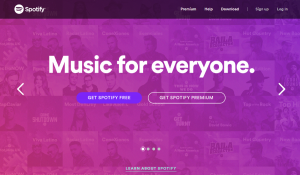The image is a compact screenshot from Spotify, predominantly featuring a purple overlay box with a black toolbar at the top. The backdrop displays slightly faded CD covers. At the top center, the toolbar displays the word "Spotify" alongside additional navigation elements. Prominently placed within the purple box is the tagline "Music for Everyone" in white text. Below this, the box offers two call-to-action buttons: "Get Spotify Free," displayed on a blue button with white text, and "Get Spotify Premium," shown on a transparent button with white text that blends with the purple background.

The bottom of the purple box features four navigation dots, followed by a link in small print that says "Learn About Spotify." In the black toolbar above, additional options appear including “Help,” “Sign Up,” and a partially readable third item, suspected to be slightly blurred. The word "Premium" is also visible at the top, reinforcing the subscription option. Overall, the graphic is straightforward, emphasizing Spotify's user options and overall theme.